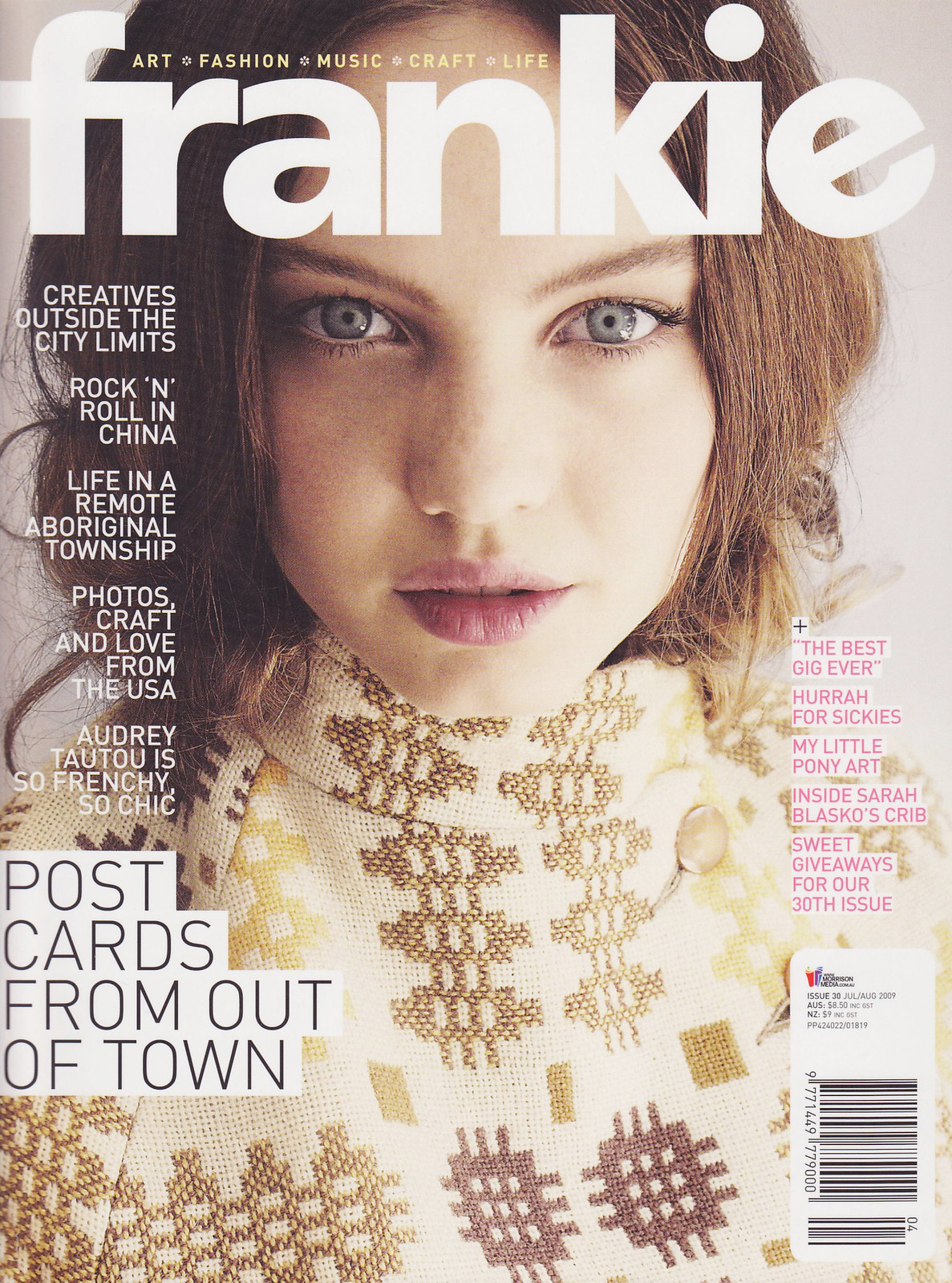This magazine cover showcases the title "Frankie" in large, lowercase white font, prominently placed over a background image of a Caucasian woman with short light brown hair and gray-blue eyes. She is dressed in a cream-colored sweater featuring a honeycomb-like pattern in variations of brown and yellow hues. Her serene expression and parted lips suggest a neutral demeanor.

Above the title "Frankie," in small yellow font, the words "art, fashion, music, craft, life" are displayed, hinting at the magazine's diverse content. Below the title, on the left-hand side, are several article headlines written in small white all-caps font: "Creatives outside the city limits," "Rock and roll in China," "Life in a remote Aboriginal township," and "Photos, craft, and love from the USA." Another headline states "Audrey Tautou is so Frenchy so chic."

In a larger black font with a white background, the headline "Postcards from out of town" appears further down on the left side. On the lower right-hand corner, there is a barcode that runs vertically. Additionally, the bottom right-hand corner features more text in pink font on a white background, advertising "The best gig ever," "Hurrah for My Little Pony art," "Inside Sarah Blasco's crib," and "Sweet giveaways for our 30th issue."